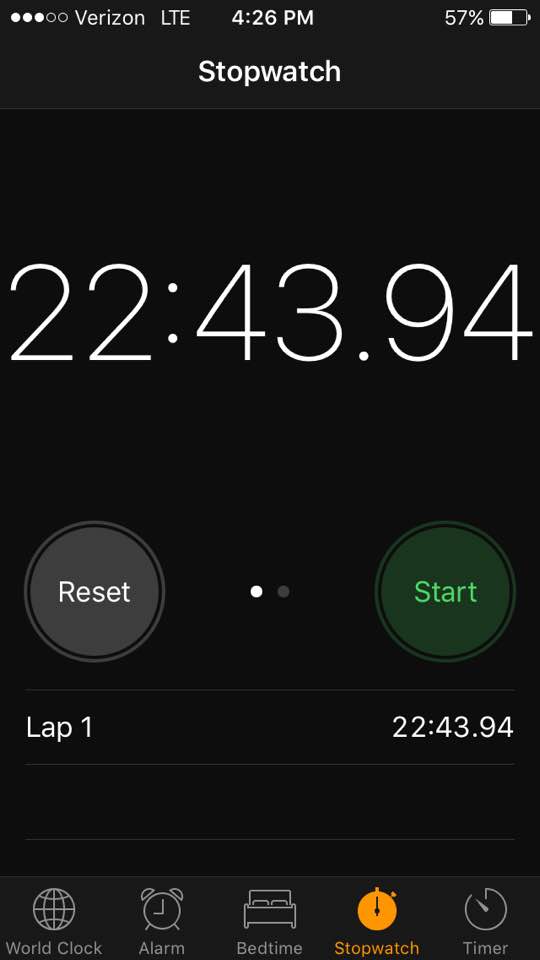This is a screenshot captured from a mobile phone displaying the stopwatch app. The background is predominantly black, with a lighter, black notification bar at the top. This bar contains essential phone details in white font, arranged from left to right: three white dots, two black dots, the word "Verizon," "LTE," the time "4:26 PM," and the battery percentage "57%" adjacent to a battery icon.

Just below the notification bar, in bold white font, the title "Stopwatch" is prominently displayed. The main screen of the stopwatch app is even darker black, with the running time shown in very large white font at the center, reading "22:43.94."

In the lower left corner, there is a gray circular button labeled "Reset" in white font. At the center bottom, there are a white dot and a gray dot side by side, likely indicating pagination. Over to the lower right corner, a brown circular button is labeled "Start" in green font.

Beneath these buttons, a gray line separates the main time display from additional information below. In white font, "Lap 1" is listed along with its corresponding time "22:43.94," followed by another gray line. The bottom of the screen features a gray bar housing four icons, whose specific details are not specified in the description.